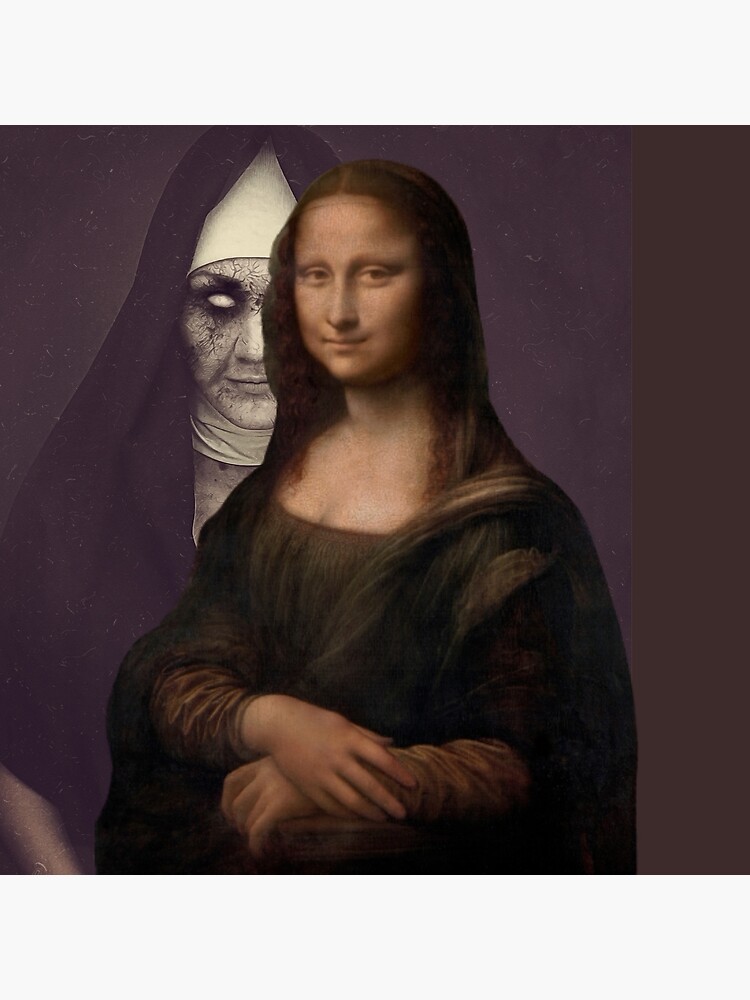This image is a spoof of the iconic painting of the Mona Lisa. The central figure is the well-known Mona Lisa, depicted with her long brunette hair, delicate fair skin, dark clothes, and almond-shaped eyes. Her hands are gracefully crossed in front of her, and she retains her enigmatic, subtle smile. The scene is set against a stark black background, but what makes this version disturbing is the figure behind her.

In the background, there is an eerie, horror-like figure dressed in black and white nun's clothing. This figure is unnervingly staring at the Mona Lisa. The "nun" has an ominous pair of eyes, with one eye appearing as a white, empty socket while the other is ringed with heavy black mascara. The face of this figure is cracked and grooved, adding to the sinister appearance. Her lips are twisted in a malevolent smile, giving the impression that she might attack the Mona Lisa. The unsettling presence of this cracked, ghostly nun peering over the Mona Lisa’s shoulder transforms the classic artwork into a scene from a horror film.